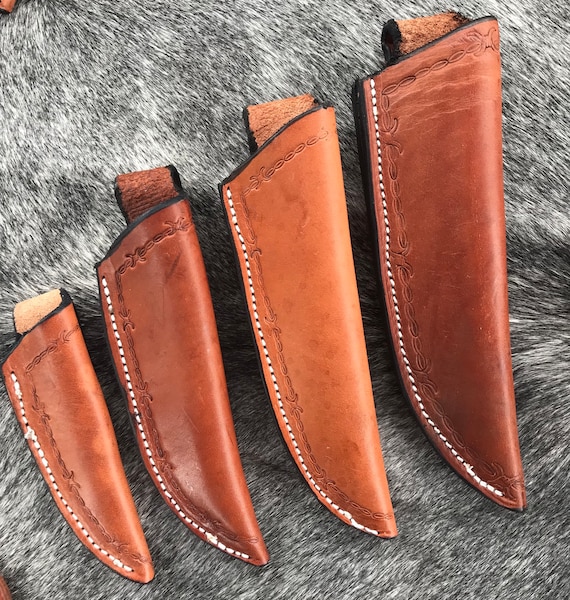The photograph showcases four leather knife sheaths arranged from left to right, increasing in size. The sheaths are crafted from brownish-orange leather with intricate white stitching, forming a barbed wire pattern along the edges. The first and third sheaths are lighter in color compared to the second and fourth, which are darker. Each sheath features a tab at the top and a holder or loop on the back for attaching to a belt. The sheaths are set against a silvery-gray, marbled fur or animal skin background, adding a textured contrast to the image.